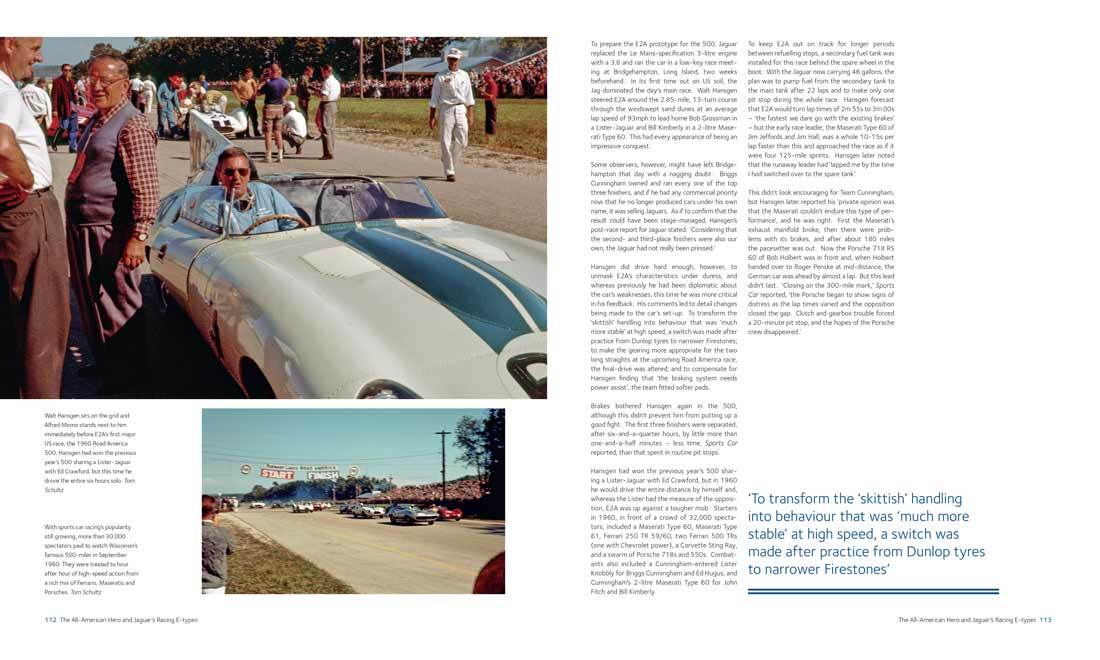The image depicts two pages from what appears to be an old magazine article. On the left page, there is a prominent photo of a man wearing a blue shirt and sunglasses, seated in a silver convertible race car with blue racing stripes. The car, likely a Shelby GT, bears the number six on its hood and is a right-hand drive model, indicating it might be of European origin, possibly from the UK given the spelling of "tyres" in the text. In the background, there are people dressed in various attires, including white clothes, brown dress pants, and shorts, going about their business near a grandstand, amidst trees, green grasses, and a house with a blue roof. Below this large photo, a smaller image shows a group of cars, varying in colors and sizes, either lined up for or actively participating in a race on a concrete road, under a clear blue sky. The right page contains the article's text in two columns, detailing, among other things, the transformation of the car’s handling through the switch from Dunlop to narrower Firestone tyres. The article is partly highlighted in blue for emphasis, with some blue writing in the lower right corner and an unreadable text possibly indicating the page number at the far bottom right.